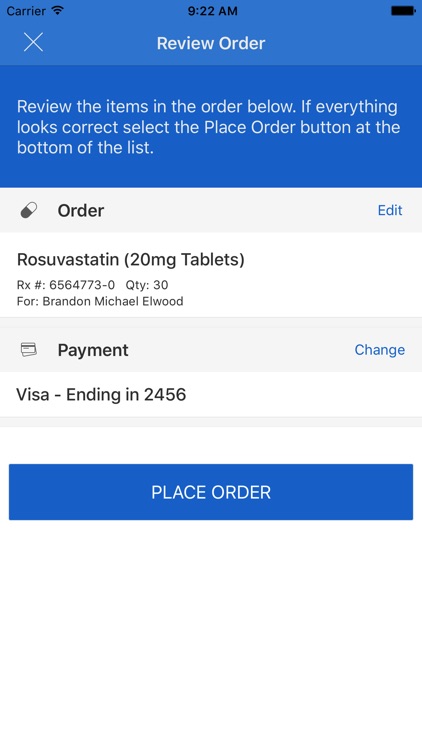This image is a screenshot capturing the review stage of an online order, presumably for a medical product. The screenshot is taken from a mobile device, evident from the phone interface displaying the time as 9:22 AM and a fully charged battery icon in the top right corner.

The image shows a page with a light blue header containing white text stating "Review Order." Directly below the header, a detailed message instructs the user to verify the items listed and to proceed by selecting the "Place Order" button at the bottom of the page.

The primary focus of the screenshot is the order information, which features a small capsule icon next to the text, indicating a purchase of medication. The medication ordered is specified as "Rosuvastatin 20mg tablets," and it is intended for a patient named Brandon Michael Elwood. The payment method displayed is a Visa card ending in 2456. 

The clean and organized layout of the page suggests the user is on a medical or pharmaceutical website, reviewing their order before finalizing it.